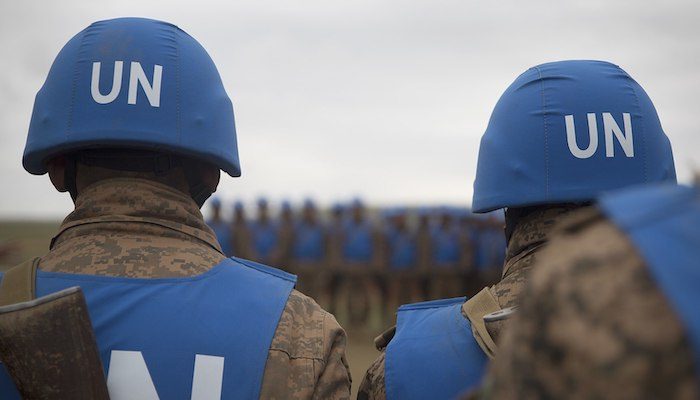In this photograph, we see an outdoor scene under a pale, gray sky, capturing a moment among United Nations soldiers. The focus is on two soldiers from the back, whose blue helmets prominently display "UN." They're also equipped with matching royal blue vests over their brown and green camouflaged uniforms. Both soldiers are standing at the ready, possibly awaiting assignment, with one carrying a well-worn wooden-handled gun strapped across his back. The scene extends to a larger formation of similarly uniformed troops in the background, blurring into a sea of blue helmets and vests. Additionally, on the left side, one soldier has a brown, rugged crossbody bag slung over his shoulder, and closer to the right edge of the frame, part of a third soldier's blue vest is visible.